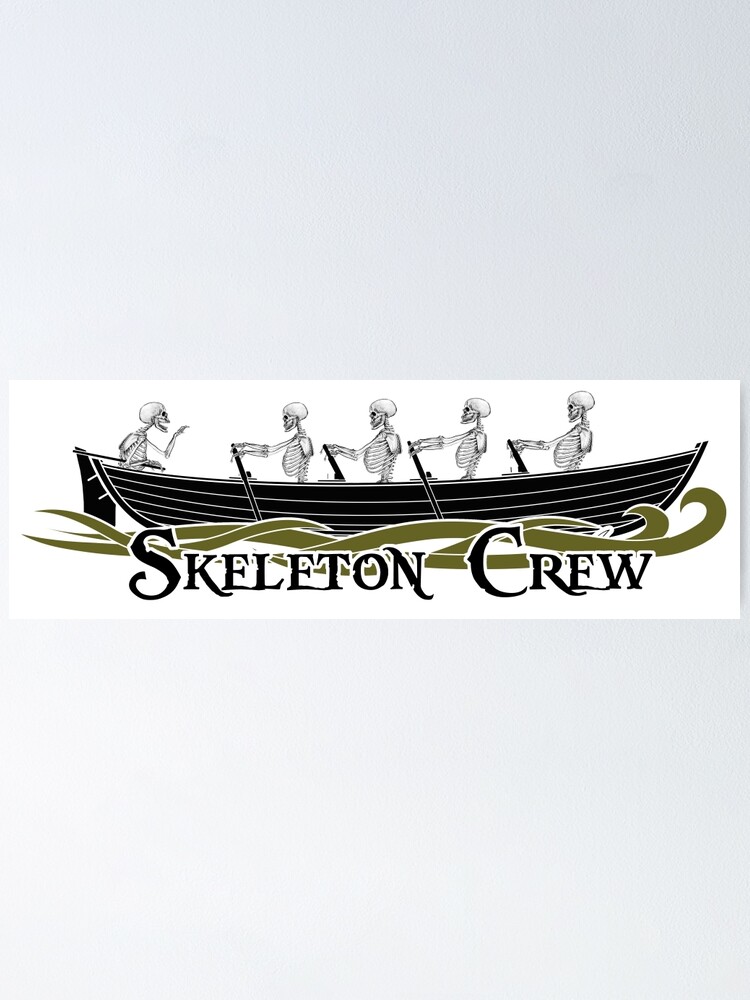The image depicts a striking piece of artwork featuring a black wooden boat with white stripes. Inside the boat, there are five skeletons rendered in simple black line art. One skeleton at the front appears to be directing the others, who are all holding oars and rowing the boat. The boat floats on an ocean subtly outlined with olive green, snake-like designs. Below the boat, the text "SKELETON CREW" is written in bold, capitalized, serif font, in a bluish color. The entire scene is set against a white background, which lies on a larger, vertically oriented dual gray rectangle.